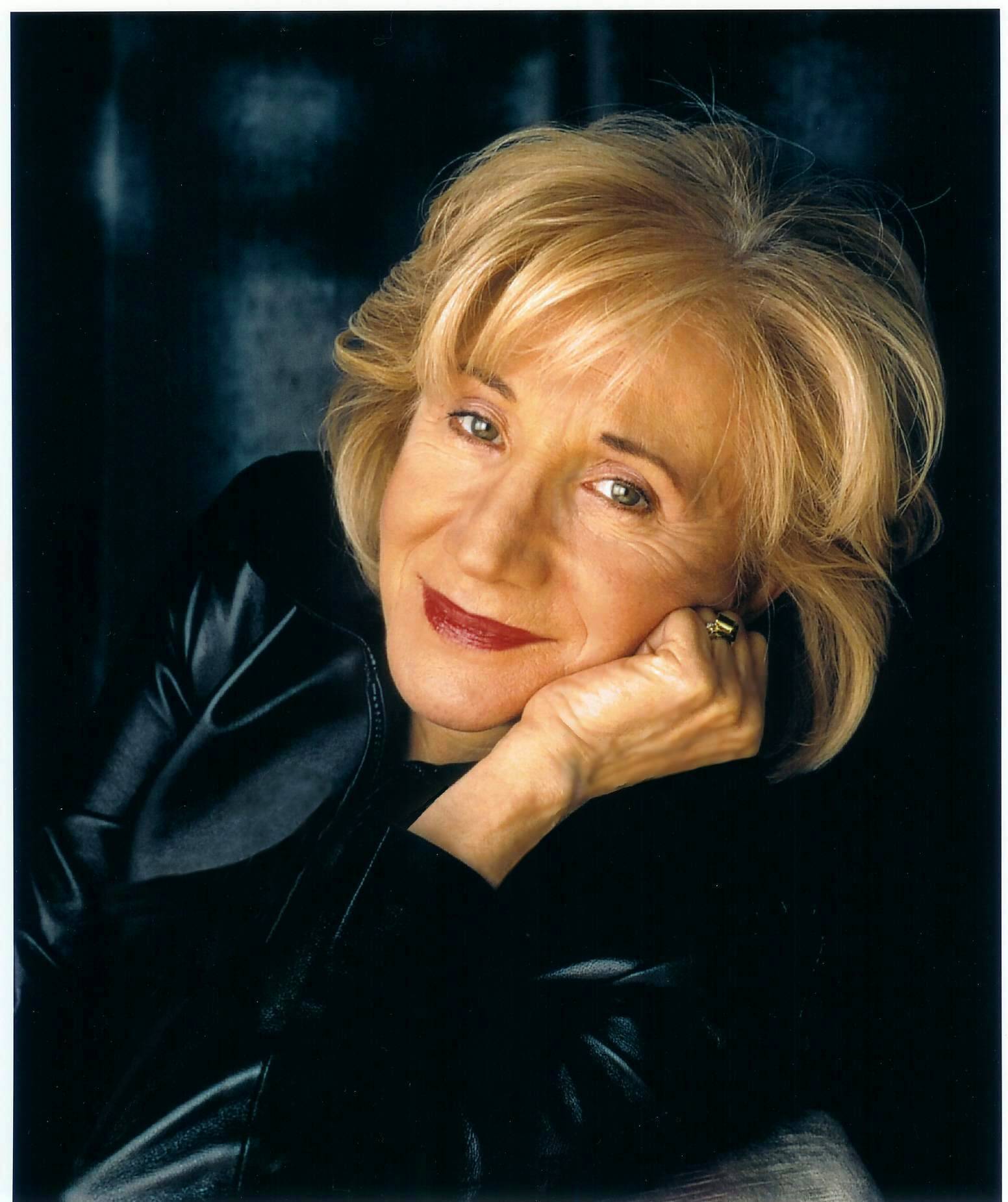The photograph is a portrait of a middle-aged Caucasian woman with short, stylishly shaggy dyed blonde hair. She is wearing a black leather jacket over a black shirt and has a gold ring on her finger. Her skin is fairly tan, and she has a warm expression in her hazel eyes. She wears bright red lipstick, and her smile is closed-mouth, conveying a friendly or wise demeanor. The woman, possibly a celebrity or public figure, is seated on a gray couch, with her left shoulder resting in the bottom right corner of the image. Her arm is bent, and her fist is propping up her head. The background features a black curtain area with muted shades blending into gray, and there are small, faded reflections around her head and shoulder. The photograph, which is vertically aligned, captures her from the torso up.